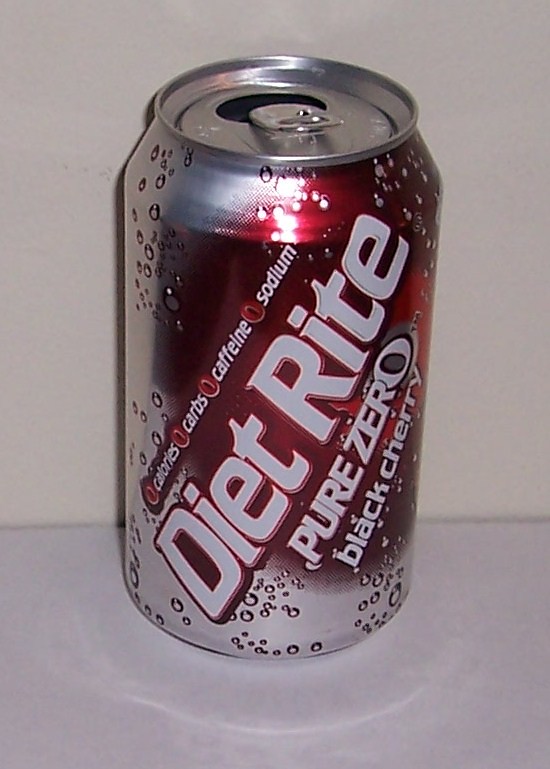A vertically framed image showcases a silver can of soda positioned at a slight downward angle. The can, which has been opened, features the tab positioned below the opening, leaving the hole prominently visible at the top. The can itself boasts a bright silver background adorned with a dark red area and numerous bubbles outlined in red. Bold white lettering reads: "Zero Calorie, Zero Carb, Zero Caffeine, Zero Sodium, Diet Rite, Pure Zero, Black Cherry."